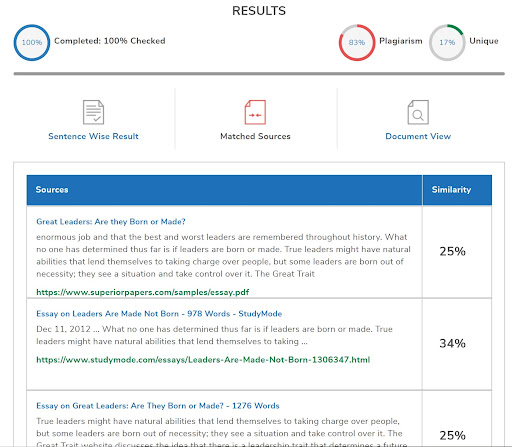This is a detailed screenshot from an undisclosed website displaying plagiarism results for a document analysis. At the top, indicators reveal "Results: 100% completed, 100% checked, 83% plagiarism, 17% unique." The interface includes tabs for "Sentence-wise result," "Matched sources," and "Document view."

Among the matched sources is a discussion on "Great leaders: Are they born or made?" highlighting the historical significance of both the best and worst leaders and questioning whether leadership qualities are inherent or developed. The document suggests that while some individuals may possess innate leadership abilities, others rise to leadership roles out of necessity, often taking control during critical situations.

The analysis cites a source from "https://www.superiorpapers.com/samples/SA.pdf" with a 25% similarity, which explores the notion that true leaders might naturally be inclined to take charge. Another referenced source is an essay titled "Leaders are Made, Not Born," consisting of 978 words, published on StudyMode on December 11, 2012, exhibiting a 34% similarity. This essay further delves into the debate, asserting that regardless of natural tendencies, effective leadership often emerges from situational demands.

The detailed view also includes a 1,276-word essay discussing whether great leaders are born or made. This essay reiterates that while some leaders have natural skills, others develop leadership qualities in response to circumstances. The content underscores the theory that a specific leadership trait might predict an individual's potential for leadership.